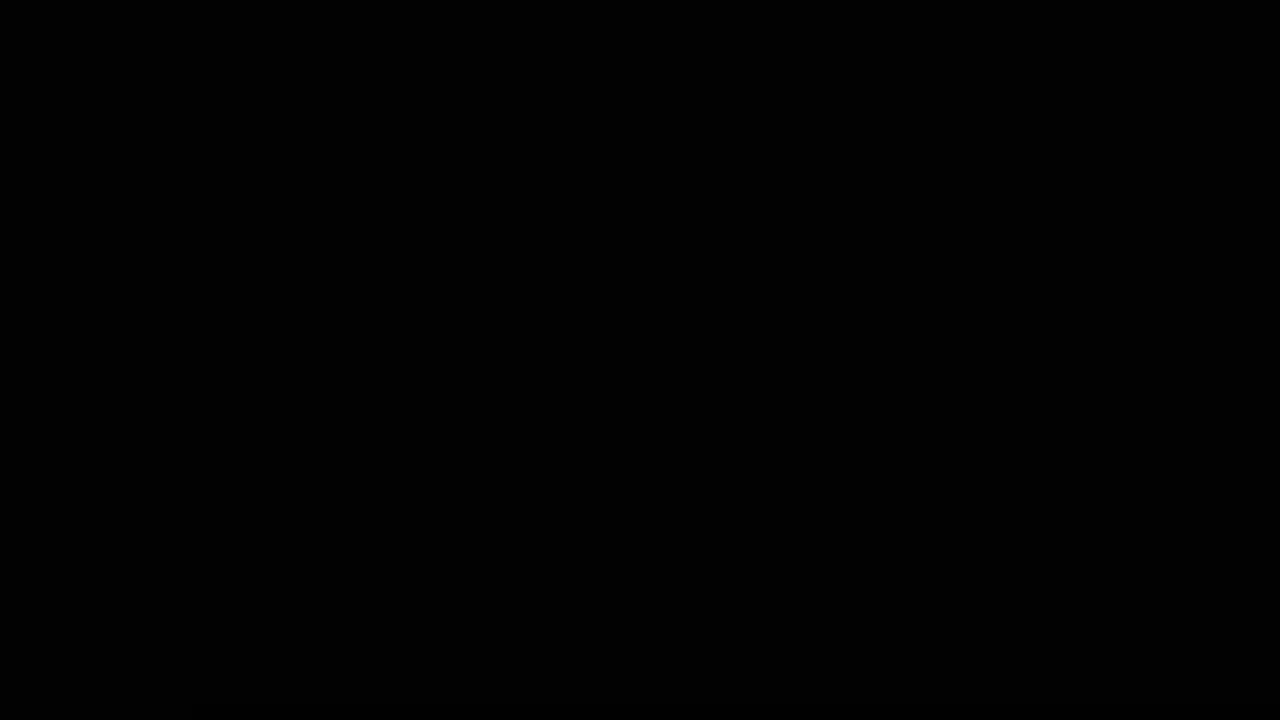The image is a completely black rectangle, occupying the entire frame with no other elements or colors present. The rectangle is horizontally oriented, meaning its length is greater than its width. The edges of the rectangle are sharp and distinct, forming precise corners. This image is a solid, pure black with no variation in shading or texture. There are no designs, objects, text, or characters within the black background, making it a stark and featureless black wallpaper. The entire image is uniformly filled with this deep black color, leaving no empty spaces or areas with different hues.